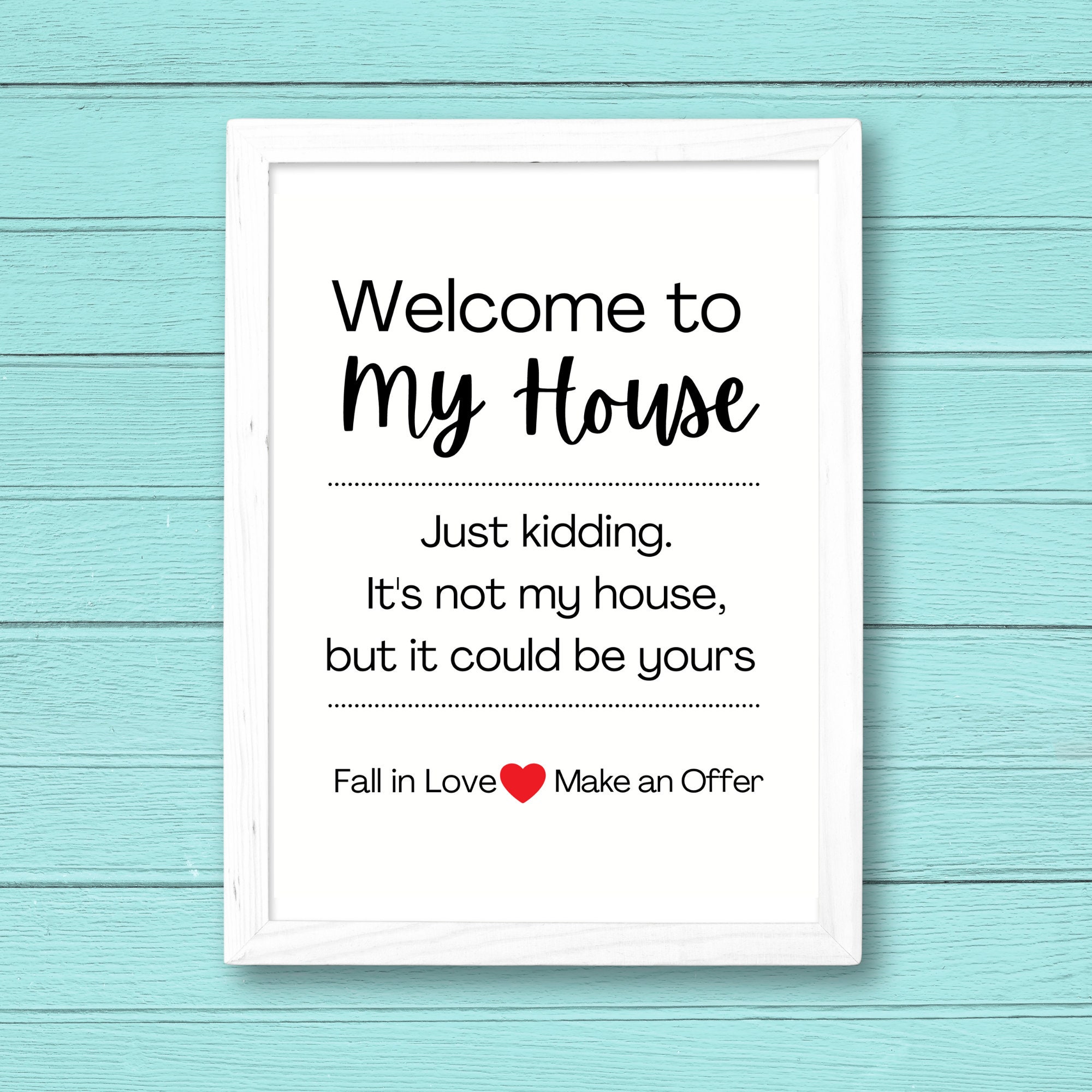This photograph features a close-up of a whimsical decorative sign mounted on a wall with teal wood paneling. The sign, which has a white rectangular frame, contains a white background with bold black text that reads, "Welcome to my house." The phrase "my house" is written in a cursive script. Below this, there is a dotted line divider followed by the text, "Just kidding, it's not my house, but it could be yours." Another dotted line divider separates this from the text at the bottom that says, "Fall in love," a red heart symbol, and "Make an offer." The entire sign exhibits a drop shadow effect, enhancing its dimensionality. The well-lit image captures the modern, tongue-in-cheek style commonly found in home decor items.